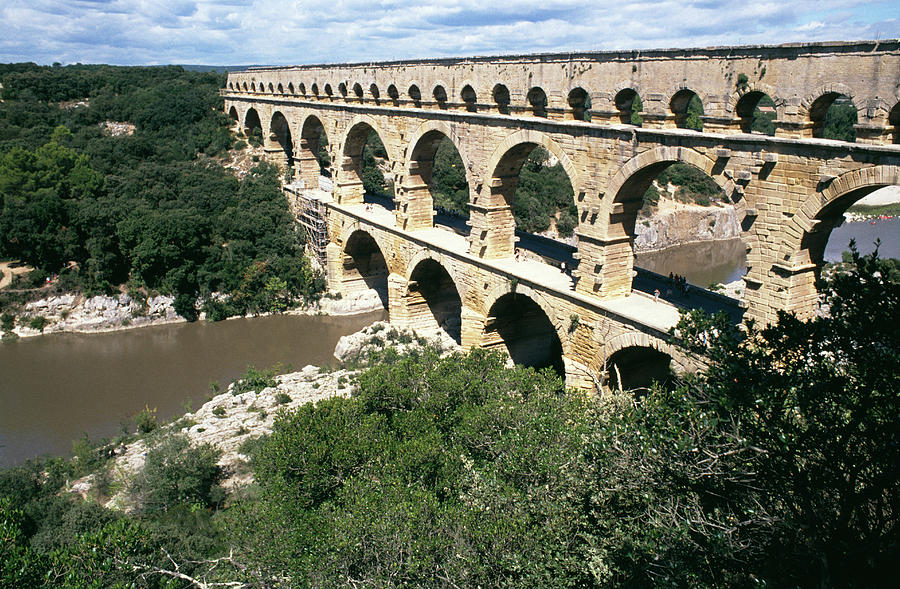This landscape photograph captures a historic double aqueduct spanning a muddy, gray-brown river that flows through a lush, forested area. The scene is framed by a narrow strip of vibrant blue sky dotted with fleecy white and darker blue clouds. The aqueduct itself, composed of light to dark brown bricks, stands prominently against a backdrop of tall, dark green trees that cover hillsides gently sloping down to the river.

The aqueduct has two main levels of archways. The upper level, stretching across the image from left to right, features around 30 archways through which the dense foliage behind can be seen. Just below this, a second row comprises about nine archways, through which the muddy river is visible, and upon closer inspection, tiny human figures can be seen walking, highlighting the structure's immense size. Near the water level, a smaller third row with about four archways is partially obscured by the river and vegetation.

Towards the lower part of the photograph, white rocks and bushy green leaves frame the riverbanks, transitioning into the dark outline of trees and undergrowth as they move toward the bottom and right edges of the image. This detailed and serene composition captures the grandeur and aged beauty of the aqueduct amidst the thriving natural landscape.